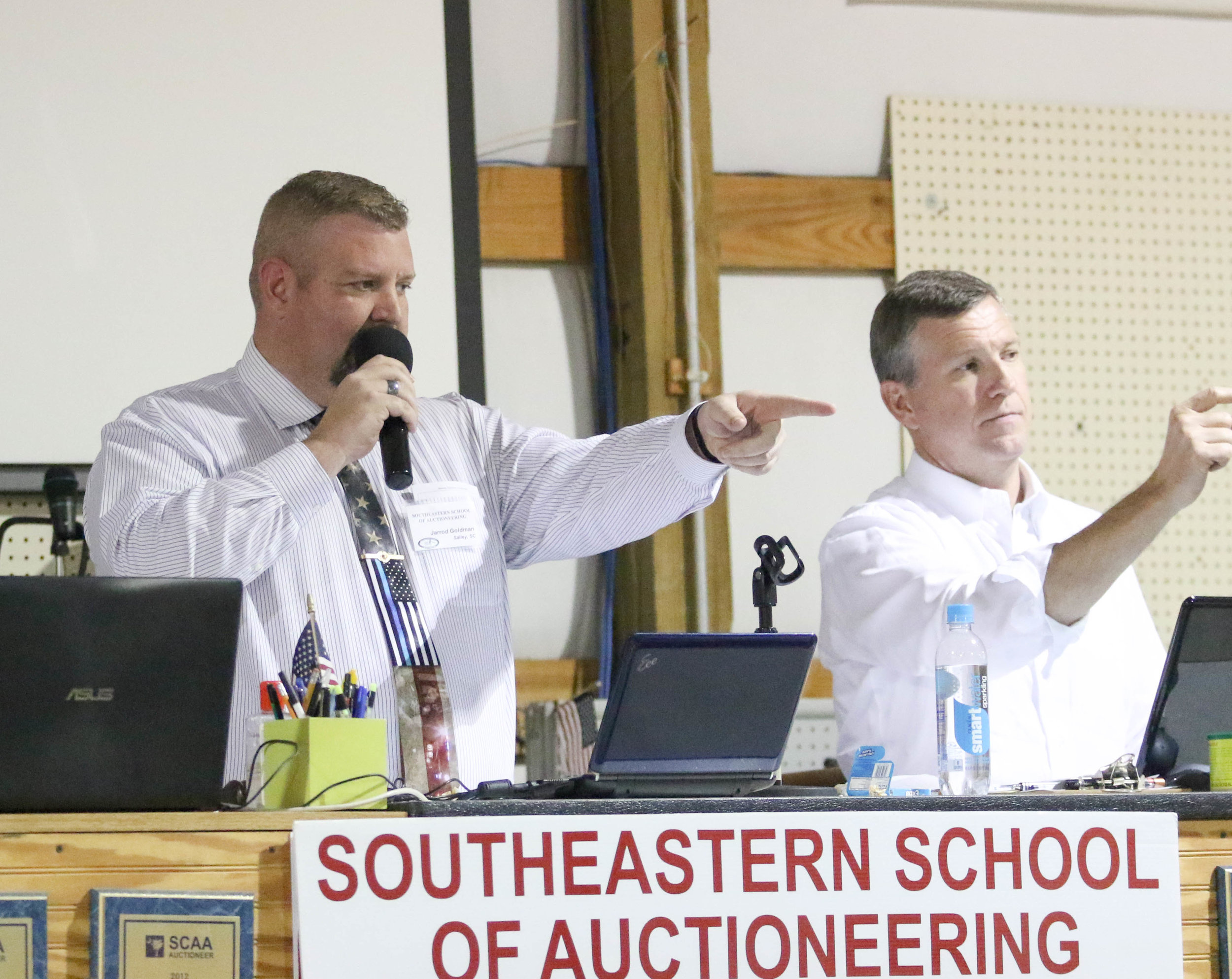The image appears to be an advertisement for the Southeastern School of Auctioneering, as indicated by the prominent text in the foreground. It features two men, likely involved in teaching or practicing auctioneering skills. The man on the right is larger, wearing a distinctive flag tie, and holding a microphone close to his mouth while pointing at something or someone. The man to his left also has his arm raised, though the exact position of his hand is unclear as it is partially cut off. They are standing behind a desk that has three open computers on top, as well as various items such as pens, pencils, and a water bottle. The scene is set indoors, with a pegboard and wooden beams visible in the background. Additionally, there are awards displayed on the front of the desk. The overall color palette of the image includes white, black, brown, off-white, red, blue, light blue, lime green, and orange. The men are centrally positioned in the image, actively engaging in what appears to be an auction.